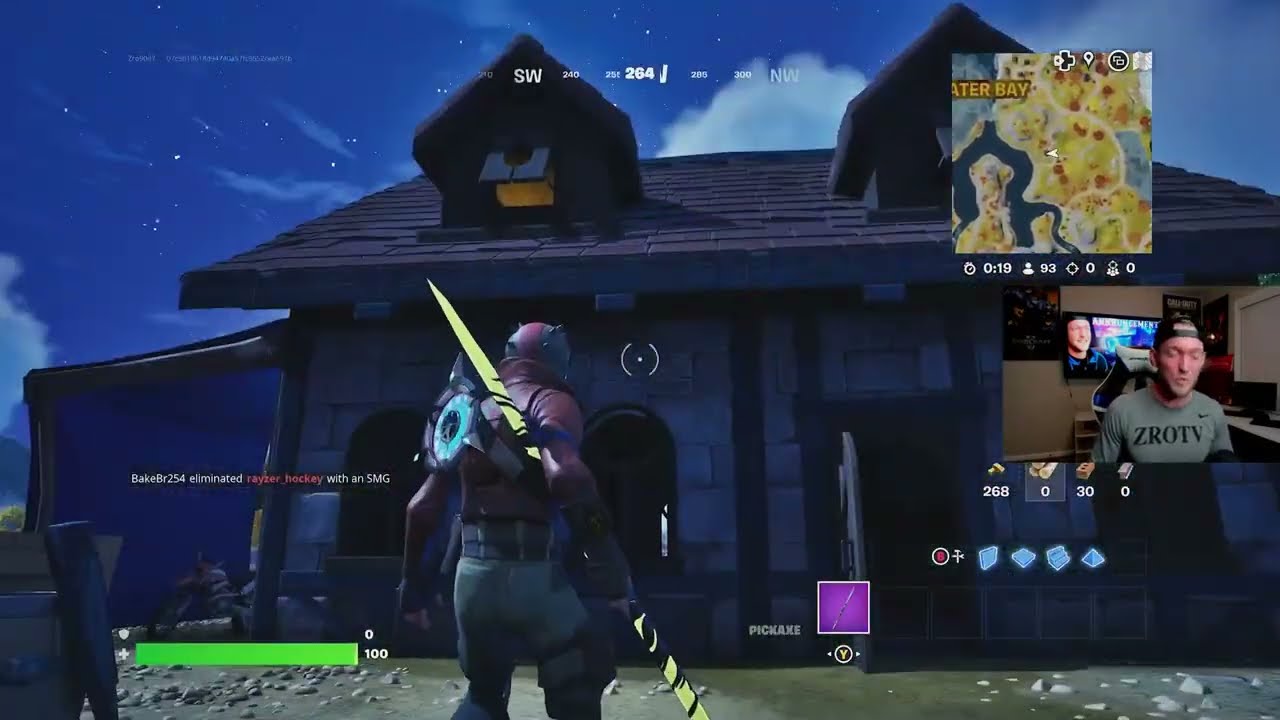This horizontal, rectangular screenshot from a video game captures an outdoor setting with a stone house featuring arched windows and an open rectangular doorway. The sky above is a dark blue with scattered white clouds. In the foreground, a character clad in red and gray armor, identifiable from the back, wields a long, light brown spear with black stripes. The character, possibly a warrior, has a purple helmet with protruding nubs and a distinctive fan-shaped, pointy-bladed apparatus attached to his back and looks as though he is walking towards the open door of the house. Near this doorway, a small purple square labeled "Pickaxe" is visible. To the upper right of the screen, there is a larger, yellow square map with white outlines and blue patches, indicating areas such as "Water Bay." On the right-hand side of the screen, there is a smaller inset image of a Caucasian man with a backward black cap and a gray ZROTV t-shirt. He appears to be playing the game shown, with a TV in the background displaying his face. The foreground display also includes certain UI elements such as a power level at 100% and various blue-hued icons.